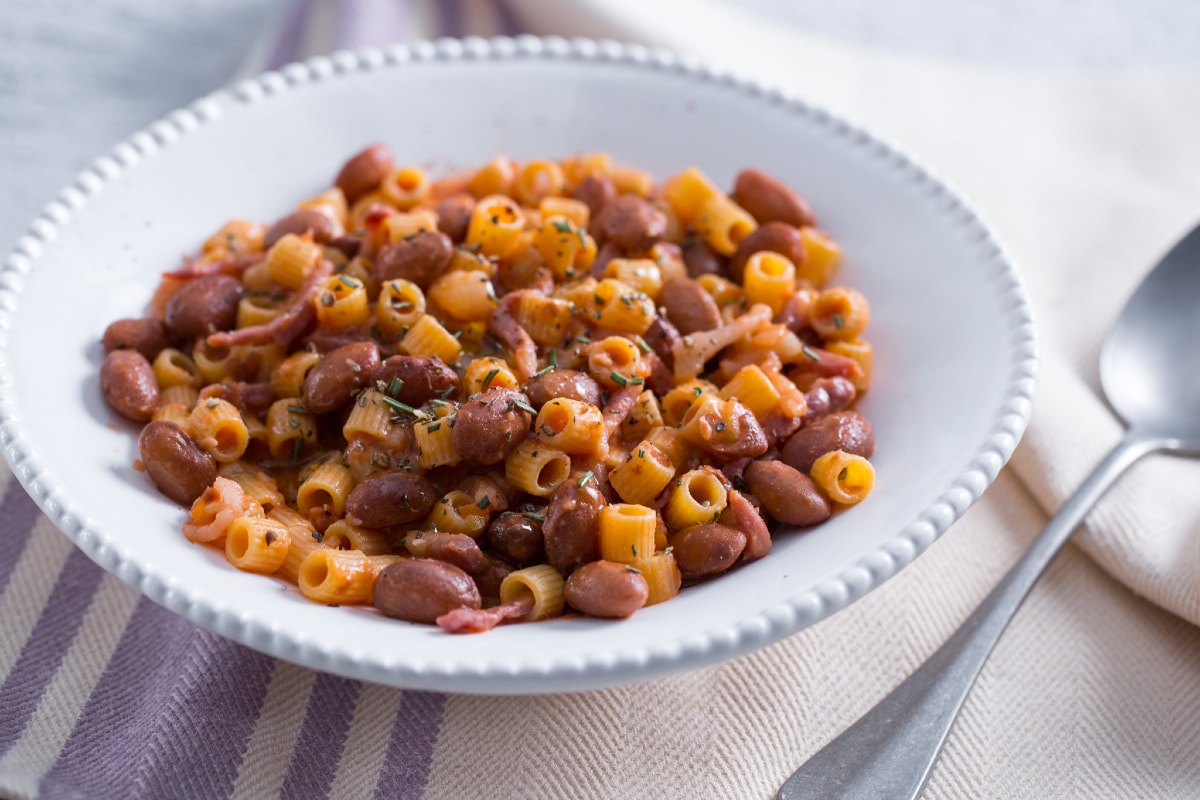The image shows a white plate with a ribbed rim, containing a dish of small, round, tubular pasta mixed with dark red or brown beans. The pasta and beans are coated in a light, possibly olive oil-based sauce, and are garnished with green herbs. The plate is placed on a predominantly white fabric with purple stripes. To the right of the plate, partially out of frame, there's a metallic spoon reflecting light.